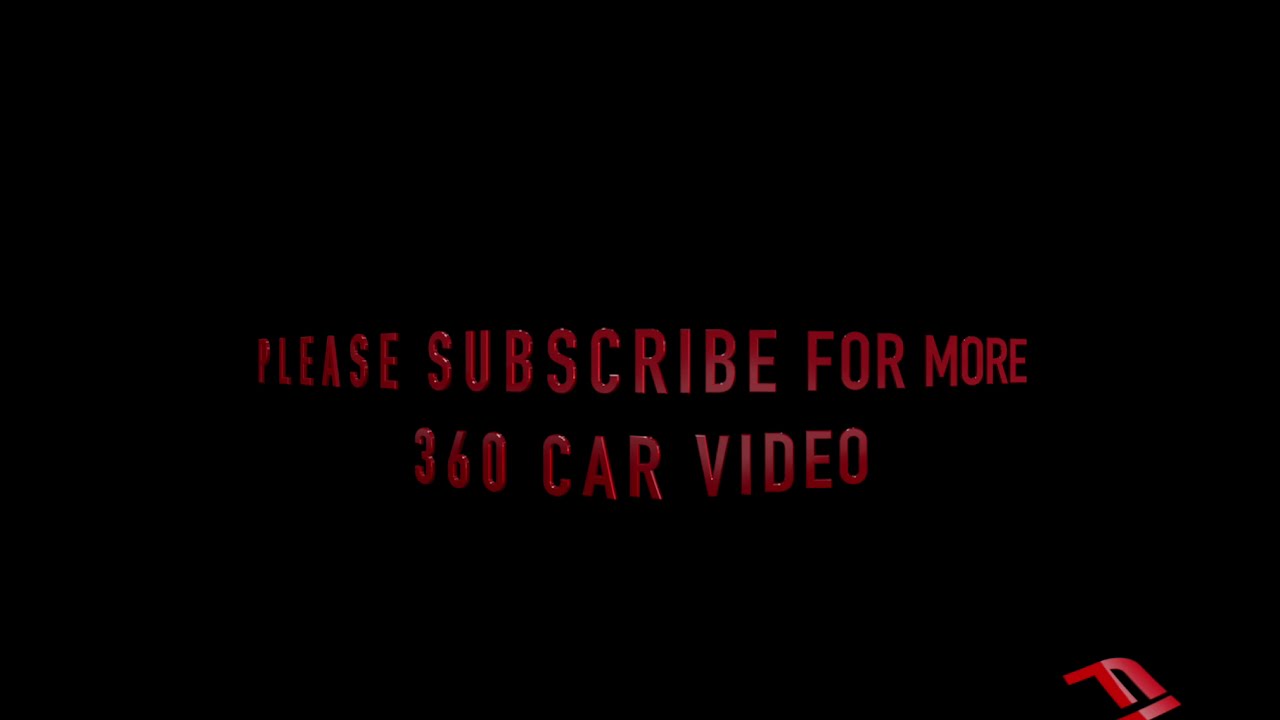The image is a promotional banner with a black background and bold red text that reads, "Please subscribe for more 360 car video." The text is split into two lines, with the words "Please subscribe for more" on the top line and "360 car video" directly underneath in slightly smaller letters. The word "subscribe" is more prominent, being larger than the other text. In the lower right-hand corner of the image, there is a red and black symbol or logo that appears to resemble a Cyrillic 'N' resting on a line or cross. The simplicity of the black background and the striking red message make the advertisement visually compelling.